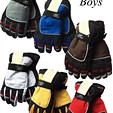This image is a small, low-resolution thumbnail, likely an ad for boys' sports gloves. The scene displays six pairs of fingerless, padded gloves arranged against a plain white background. Each pair has a different color accent, covering the palm and part of the fingers, with a consistent black color on the fingertips, wrist area, and back. Starting from the top left and proceeding to the bottom right in a diagonal line, the colors are arranged as follows: gray and black, blue and black, brown and black, white and black, yellow and black, and red and black. In the top right corner, partially cut off, is the text "BOYS" in black, indicating the target demographic. These gloves appear to be designed for activities like baseball, skiing, or golf, featuring velcro closures for a secure fit.